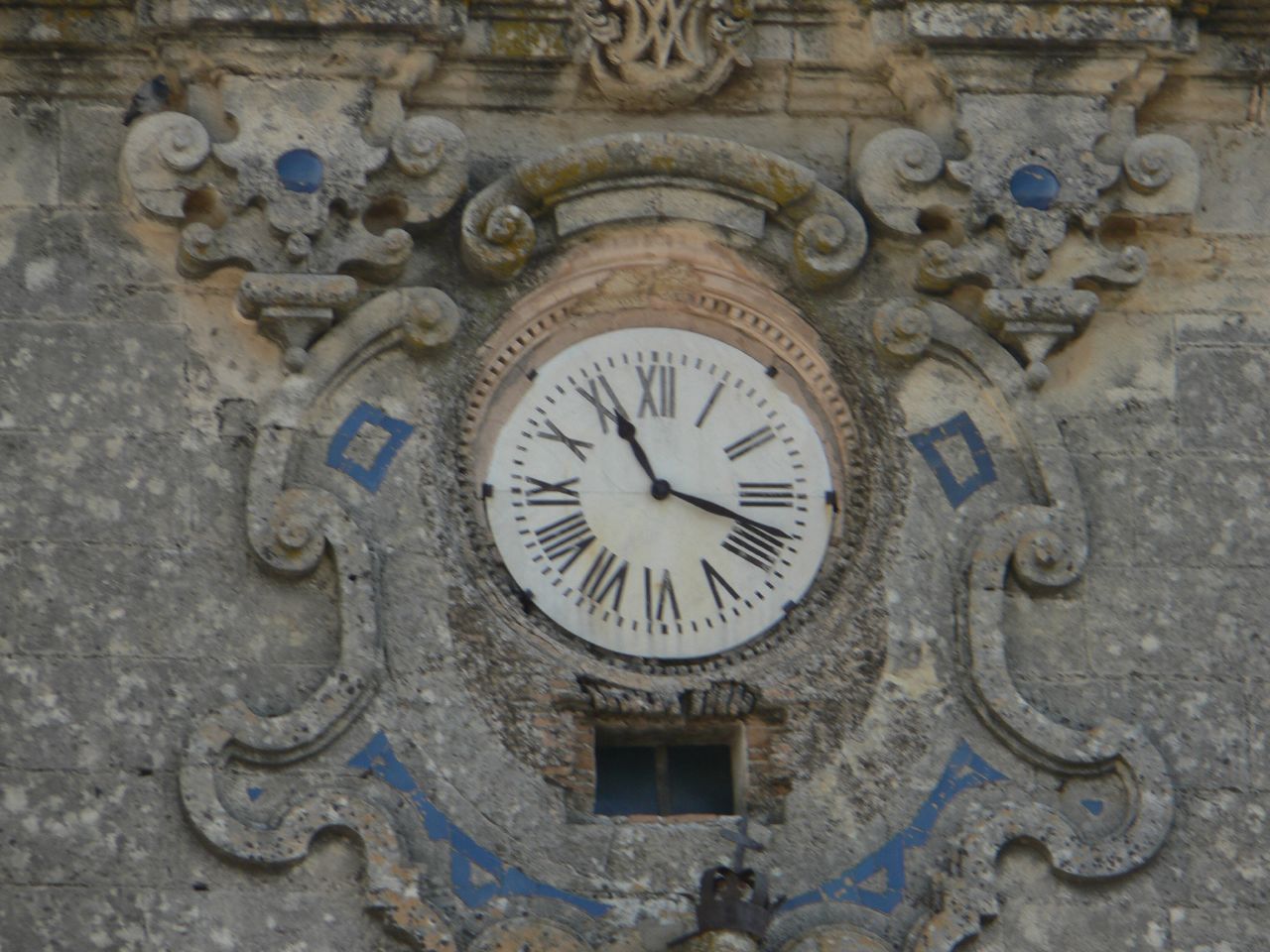This photograph captures an intricately carved stone building featuring a centrally positioned, round clock face with Roman numerals, currently displaying 11:18. The clock, encased in a gray stone carving, is adorned with small, square-like black prongs along its left and right sides, securing it to the elaborate stonework. Below the clock, a very small, rectangular window is seamlessly integrated into the stone. A rusted metal rod, possibly part of a chime mechanism, is visible near this window. Enhancing the elaborate carvings are blue square accents angled towards the top left and top right of the clock, as well as a blue semicircular banner at the bottom, resembling a smile. The center of the stone carvings, surrounding the clock, mimics the shape of a shield, embellished with complex swirls and pointed details, showcasing the artistry and craftsmanship involved in the building’s design.